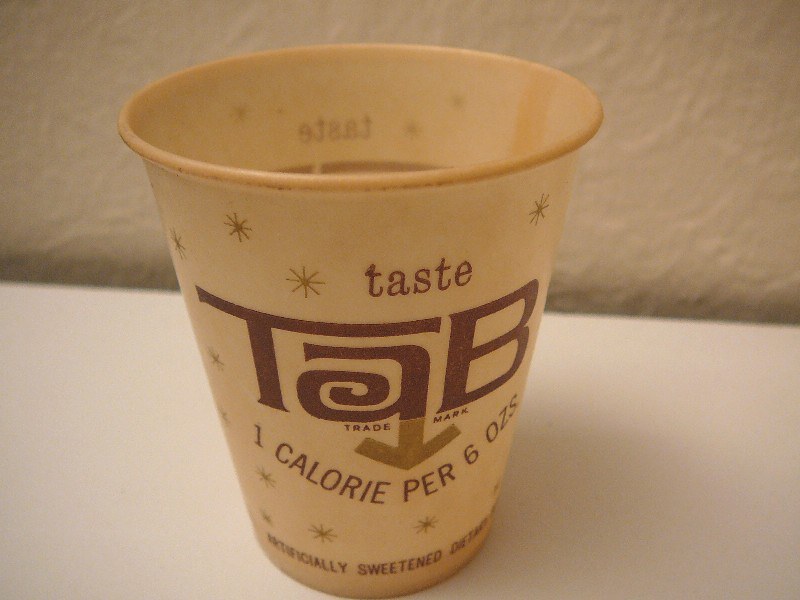The image depicts a cup with a vintage design, prominently featuring a logo that reads "Taste TAB™." The cup, in shades of off-white and tan, looks as though it has been stained by coffee or tea over time, giving it a well-loved appearance. Below the word "TAB," in a brown font, the cup states "one calorie per six ounces," and further down, it mentions "artificially sweetened," though the text is partially obscured. The design also includes small, star-like shapes scattered around the text. The cup is placed on a white shelf, which contrasts with the textured white wall in the background, emphasizing the cup as the focal point of the image.